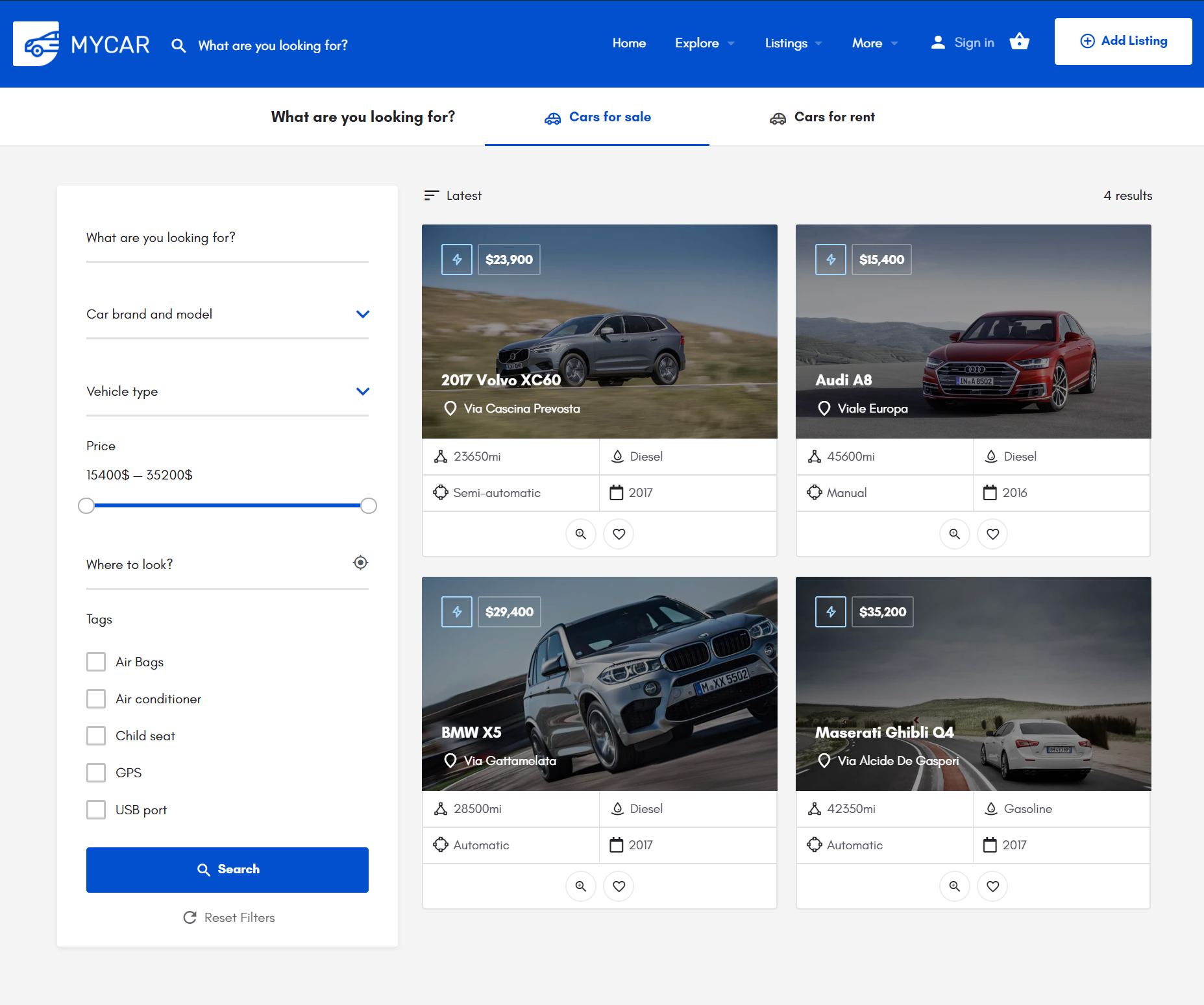The image showcases a car shopping website, displaying a selection of vehicles available for purchase. In the top left corner, the site offers navigation options, including links to the home page, car listings, sign-in, and cart functionalities. An advertisement appears on the far right side of the page. The main content shows several cars for sale, with detailed descriptions and prices.

- **Main Listings:**
  - A 2017 Volvo XC60 priced at $23,900.
  - An Audi listed for $15,400.
  - A BMW X5 available for $29,400.
  - A Maserati Ghibli Q4 shown for $35,200.

The sidebar menu provides various filters to refine the search by car brand and model, vehicle type, price range, and features such as airbags, air-conditioning, and GPS. All vehicles listed appear to be in excellent condition, highlighting the website's dedication to showcasing well-maintained cars for potential buyers.